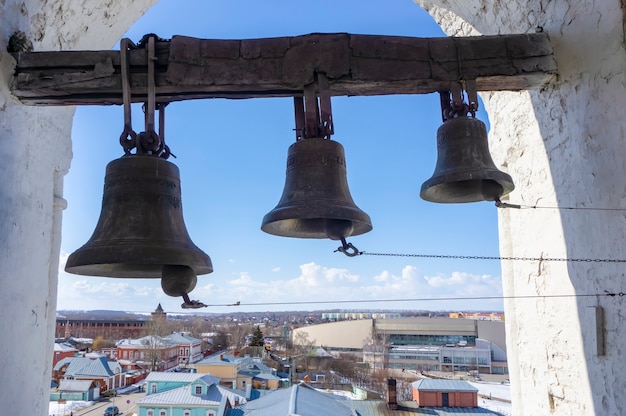In this image, three cast iron church bells of differing sizes hang from a long wooden beam that spans a white-painted brick archway. The largest bell is positioned on the left, followed by a medium-sized bell in the center, and a smaller bell on the right. Each bell is connected to a long string, extending horizontally to the right, which allows them to be rung. The background reveals a quaint older European cityscape, with several buildings, streets, and a performing arts center. Above, the sky is partly clear with cumulus clouds scattered across it. Distant mountains add depth to the scene, creating a picturesque and serene setting. The overall ambience suggests a historic and possibly significant location, where these bells may have once played a central role in the community.